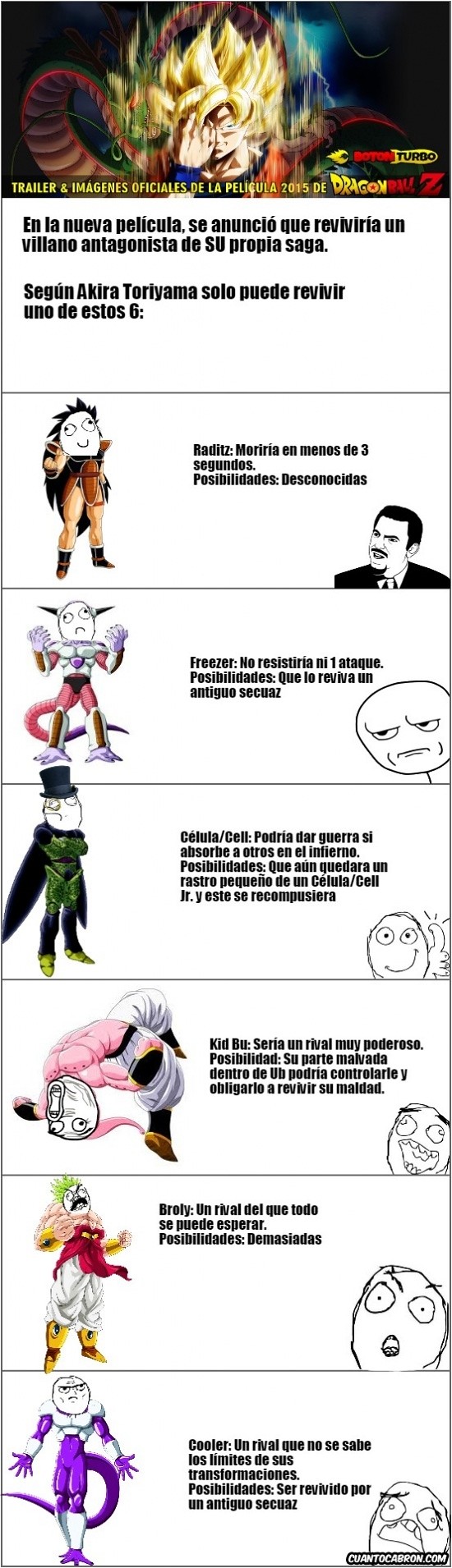The image is a screencap meme featuring a vertically stacked arrangement of characters from the Dragon Ball Z series, particularly focusing on the DBS Broly arc. The top section prominently displays Goku with his signature tall, spiky blonde hair, looking serious with one hand over his face. Behind him, the majestic green dragon Shinran snakes around, partially obscured but visible with some brown scales. The iconic Dragon Ball Z logo, in a blend of yellow and red, is present but partially hidden by additional yellow text. Below this, the meme, captioned in Spanish, comprises six smaller panels. The panels depict various Dragon Ball Z characters, including Raditz, Frieza, Cell, Kid Buu, Broly, and Cooler, but with humorous, exaggerated faces commonly used in internet memes. The text in these panels is small and also in Spanish, adding to the overall playful and comedic tone of the meme.